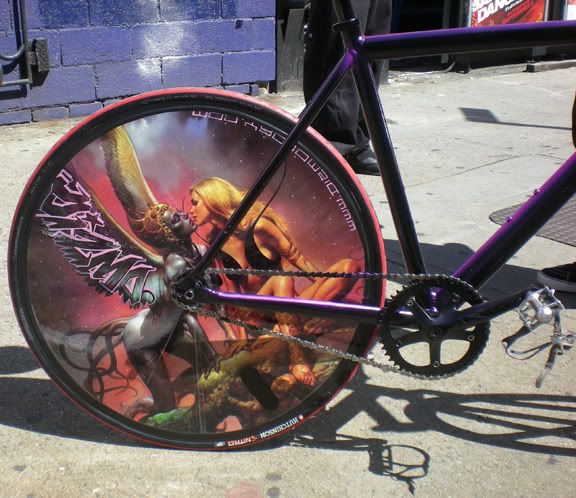In this image, we see a bicycle wheel featuring an intricate and imaginative artwork positioned behind the spokes. The artwork depicts a dynamic scene, dominated by a central female figure who evokes the essence of a warrior akin to Xena. She is dressed in black active wear, with her toned arms and legs prominently displayed, one of which bears an upper armband. Her blonde hair cascades around her as she exudes strength and grace.

Adjacent to her, a small, fairy-like figure with delicate gray wings appears to be ascending towards her. This winged being seems intent on delivering a gentle kiss to the warrior-like lady. The artwork includes a few cryptic elements, such as the letters "ZMA," woven into the design, suggesting a hidden message. The fusion of these elements transforms the bicycle wheel into a unique and captivating piece of art, making a bold visual statement.